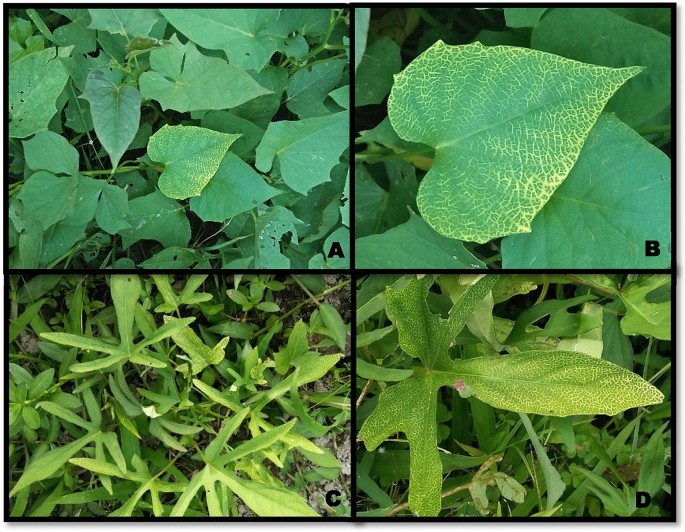This image features four distinct types of leaves organized into four labeled panels (A, B, C, and D), each showcasing a unique leaf structure. 

**Panel A, located at the top left, displays spade-shaped, heart-like leaves with smooth, dark green surfaces. Some leaves show holes or spots, adding to their natural appearance.**

**Panel B, the top right, presents a close-up of a leaf similar to A, highlighting its sharp-pointed edges and intermingling green and yellow hues.**

**Panel C, situated at the bottom left, features slender, long leaves resembling arugula, contributing to a grassy, star-like formation with five distinct points on each leaf.**

**Panel D, the bottom right, mirrors Panel C with a zoomed-in view, providing a closer look at its intricate leaf structure and a small purple flower growing among it.**

Each photograph is set against a backdrop of dense, overlapping vines and foliage, with the ground partially visible, revealing a mix of mulch, dirt, gravel, and white sand. The labels are in dark, bold lettering, enhancing the clarity and organization of the imagery. The entire scene captures the vibrant, diverse beauty of natural leaf patterns in a well-detailed, quad-panel format.